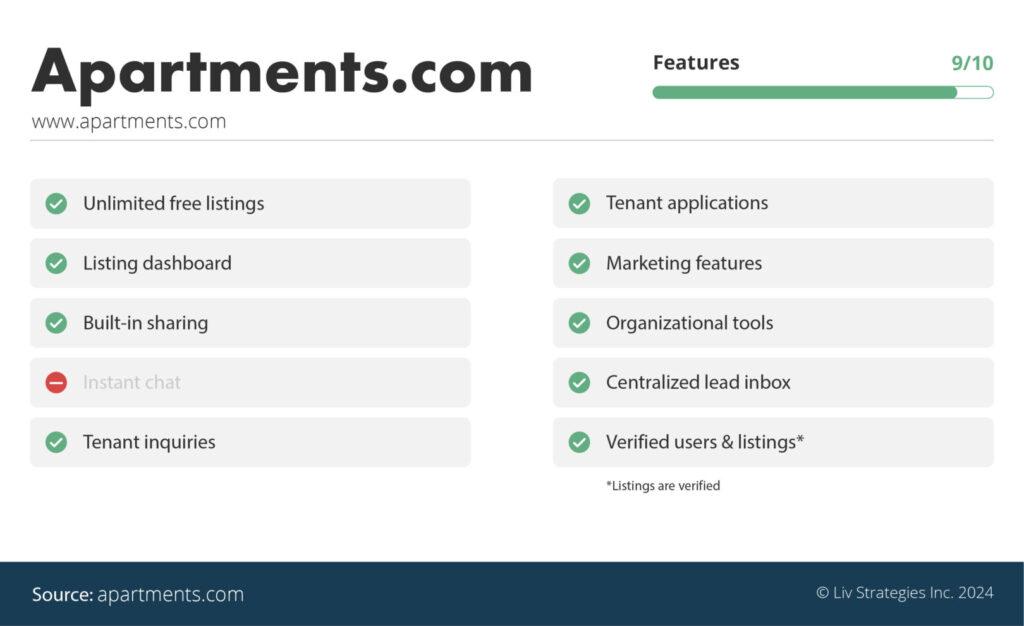This image is a screenshot of the Apartments.com website. On the left side, the text "Apartments.com" is prominently displayed in bold black font. Below this, the website address, "www.apartments.com," is repeated in dark gray text. 

On the right side of the image, various available features are listed, rated 9 out of 10 in green text. Below this rating, a progress bar visually depicting 90% completion is displayed in green. The included features are marked with green circular icons with white checkmarks, while excluded features have red circular icons with white slashes.

The included features are:
- Unlimited Free Listings
- Listing Dashboard
- Built-in Sharing
- Tenant Inquiries
- Tenant Applications
- Marketing Features
- Organizational Tools
- Centralized Lead Inbox
- Verified Users and Listings

The only feature not included is labeled "Instant Chat."

At the bottom of the image, a source label "Apartments.com" is placed on a dark blue rectangular background. Additionally, copyright information is visible on the right side, written in light blue text.